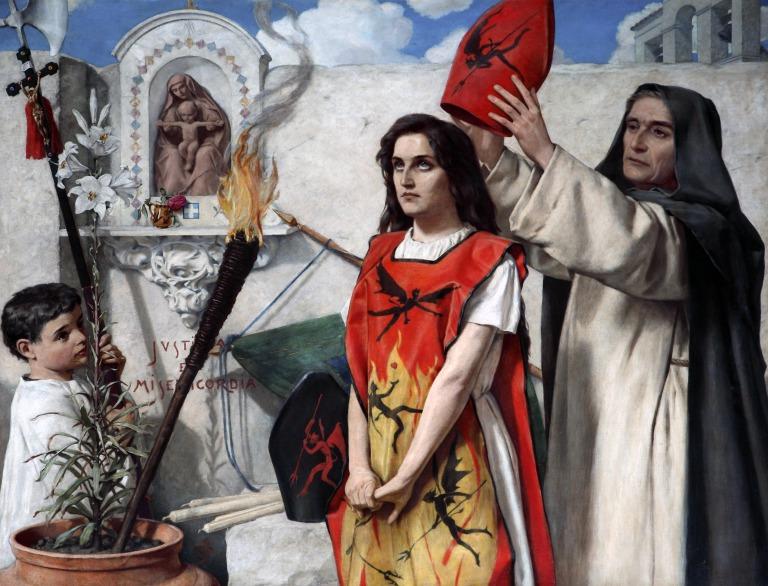In this intricately detailed artwork depicting a religious ceremony, the scene is set within a white stone area under a bright blue sky dotted with white clouds. The focal point of the image is a young Caucasian woman, likely in her early 20s, who stands at the center. She wears a white underdress paired with a distinctive red apron adorned with black and yellow angelic or demonic figures, with flames rising from the bottom. Upon her head, an older woman with gray hair, dressed in a green robe over a white underrobe, is placing a red hat which also features similar angelic or demonic imagery.

To the right of the scene, another figure, dressed in a white robe with a black cowl, stands, contributing to the ceremonial atmosphere. On the left hand side, a young boy, also in a white robe, holds an elaborate staff adorned with a cross and crucifixion imagery, possibly suggesting his role as an acolyte. Next to him, there is a potted plant with a torch emerging from it. Additionally, in the background to the left, an arch reveals a brown-colored depiction of a woman and a young boy, perhaps a statue of Mary with the baby Jesus. Above them, dark gray arches create a striking contrast against the serene sky. This rich tableau conveys a moment of significant religious import, possibly a canonization or a bishop’s consecration.